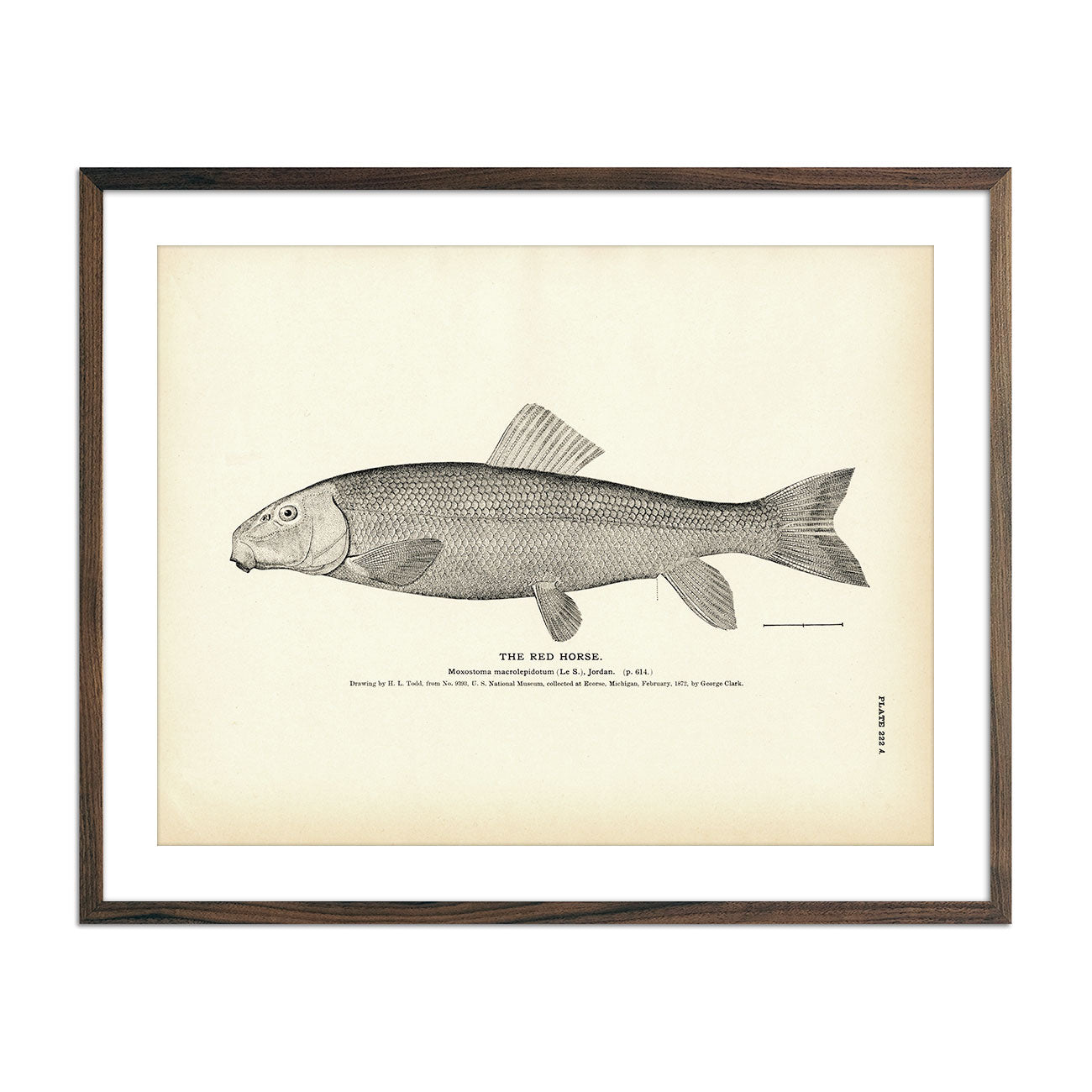This framed and matted line drawing, in a brown frame with white matting, features a detailed profile sketch of a fish labeled "The Red Horse." The artwork is rendered in shades of gray on an off-white background, with intricate lines highlighting the fish's scales and fins. The fish has a prominent, slightly downward-pointing mouth, a large eye, a small dorsal fin, and multiple side fins, with one distinctly visible fin on the opposite side. The legend "The Red Horse" is printed in black beneath the fish, accompanied by smaller, illegible text. Additionally, the notation "plate 222A" is found on the bottom right-hand side, adding a touch of scientific or artistic classification to the piece.